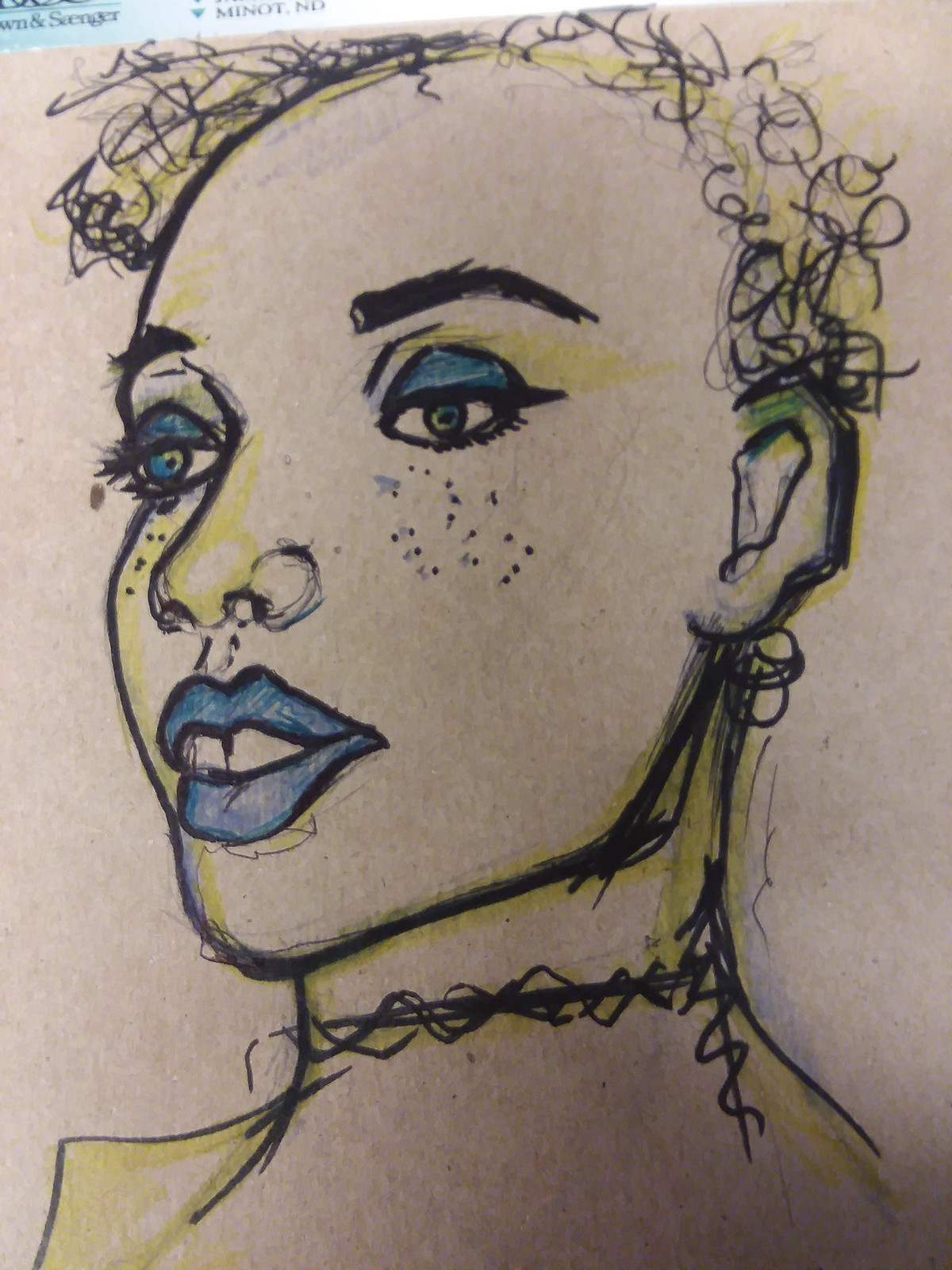In the illustrated image, a person is depicted looking down towards the left with an expression of contemplation. The artwork is created using a combination of pen and markers. The individual features wiry, curly hair, giving them a distinctive and textured appearance. Their left eye is adorned with blue eyeshadow and is vividly blue itself, accentuated by a thick eyebrow. In contrast, the right eye has a yellow hue, with a blue eyelid and a green iris, set against a white background. Both eyes are surrounded by freckles, adding to the character's unique look.

The nose has a slight yellow tint, while the lips are colored light blue with a bold black outline. The facial features and the head are primarily outlined in black, adding definition to the illustration. The person is wearing a neck collar or a choker that is intricately designed with lines and swirls, adding an element of fashion and detail. There are also areas of yellow on both the left and right sides of the image, contributing to the overall vibrant and eclectic style of the artwork.